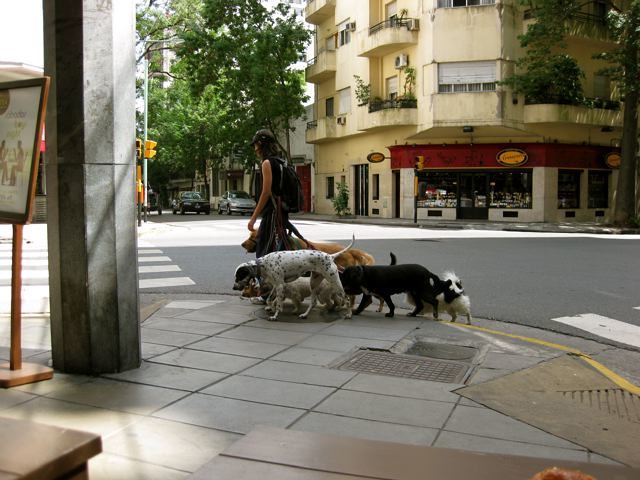In this detailed image, a woman is prominently walking five to six leashed dogs along an urban sidewalk. She is positioned centrally in the frame, moving towards the left side. The woman, distinguishable by her black cap, sleeveless black shirt, rucksack, and sunglasses, holds the varied pack close together. Among the dogs, there is a medium-sized golden retriever, a black dog of similar size, a spotted black and white dog, a small predominantly white dog with a brown head, and another small black and white dog. The background features a bustling cityscape with a storefront on the ground level of a building that appears to have apartments above it. Trees line the opposite side of the street, and a column with a display to the left suggests the photograph was taken from inside a restaurant. Additional urban elements such as a zebra crossing, traffic lights, and distant cars also contribute to the scene. The street, devoid of other pedestrians, amplifies the focus on the woman and her dogs.